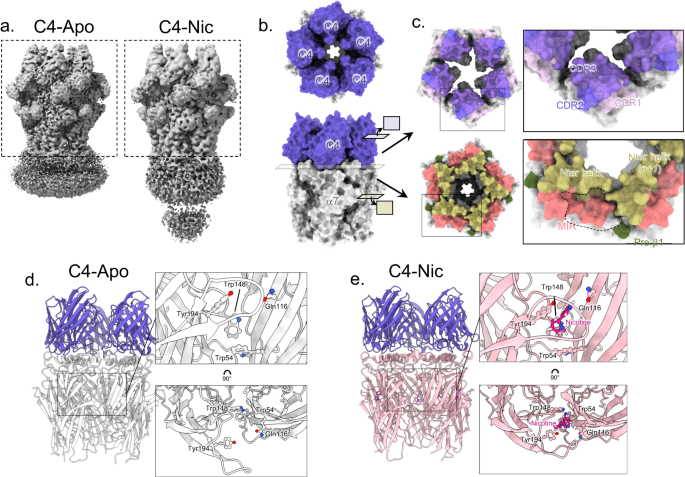The image features an array of vibrant flowers in a variety of colors, including purple, pink, and yellow. These flowers, arranged in a circular formation, create a striking contrast against the solid white background. The scene is further divided into five sections labeled A, B, C, D, and E, with each section displaying artistic elements that resemble microscopic structures. Among these elements are colorful silver, purple, pink, and yellow blobs, and gray, purple, and pink ribbon-like forms. Across the composition, repeated text such as "C4APO" and "C4NIC" appears, adding to the intricate design. The overall effect is a visually captivating blend of vibrant florals and detailed, abstract patterns.